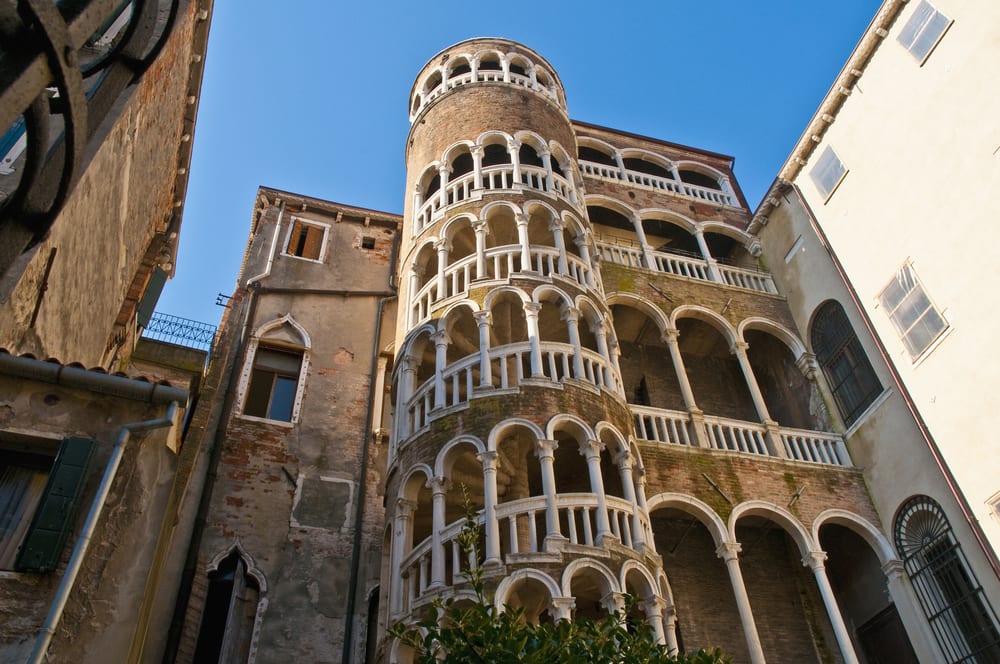The image captures a striking, tall building, possibly dating back to the 1800s or early 1900s, and appears to be located in Italy. The towering structure, constructed from taupe-colored brick, showcases exquisite architecture reminiscent of the Coliseum, featuring a prominent, spiral staircase adorned with off-white arches that frame each step. This staircase is positioned centrally, ascending gracefully and drawing the viewer's eye upwards. The sky is a vivid blue, enhancing the building's majestic presence.

To the right of the spiral staircase, the building is decorated with several archways that diminish in size as they ascend towards the top, adding a dynamic visual rhythm to the facade. Meanwhile, the left side presents a more austere appearance with a less detailed wall, marked by old bricks and fewer archways. At the left edge of the building, a fence can be observed.

The structure stands amidst a cluster of other buildings, possibly enveloping a courtyard, with varied window designs including pointed arches and rectangular forms. There is also a balcony on the right framed with small white arches and a solid balustrade. The intricate details of the pillars and archways emphasize the building's historical and cultural significance, making it a focal point suitable for a travel magazine or blog.